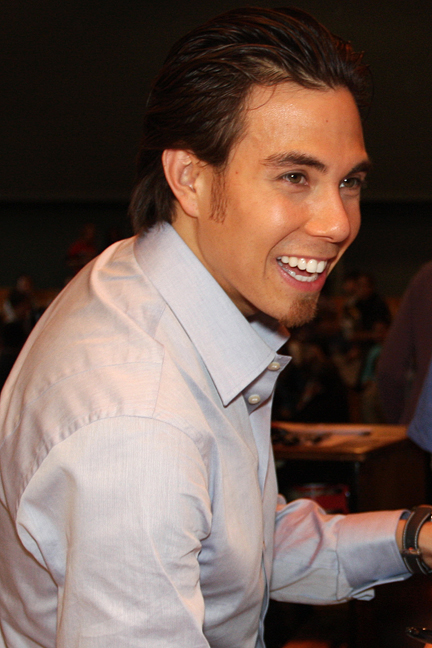In this image, a young tan man with slicked-back dark brown hair and a slight goatee gazes forward with a warm smile, revealing his teeth. He is wearing a light blue, closely paired with a whitish-gray, collared shirt with long sleeves, buttoned almost to his neck but leaving a few buttons undone. A black wristband adorns his wrist. His sideburns extend down to his jawline. The background is quite dark and somewhat blurry, featuring a black wall, and faint outlines of people seated at tables, with a wooden table noticeable on the side. The focus is sharp and clear on the man, suggesting the use of a camera flash, while the hazy backdrop amplifies his prominence in the photo.